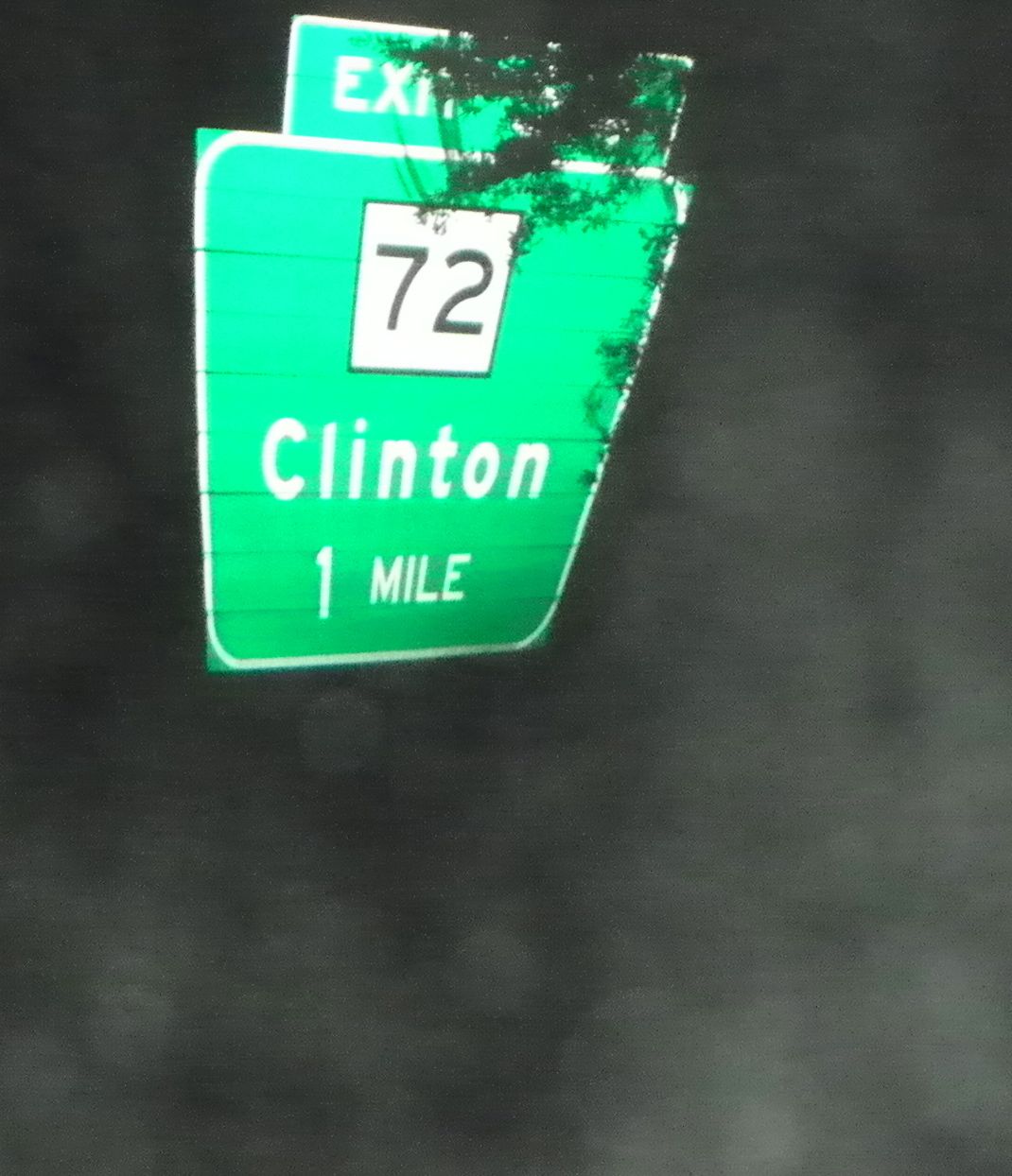In this semi close-up photograph taken at night, we see a green highway sign with a blurry mottled gray, white, and black background. The sign itself comprises two sections: a larger green square and a smaller horizontal rectangle above it. The entire sign is outlined in white. In the center of the square section, there is a white square outlined in black, containing the number "72" written in black letters. Below this, the word "Clinton" is displayed in white letters with "1 mile" indicated beneath it. The rectangular section at the top reads "EX" in white letters on the left side, but the rest is obscured by a black patch, which could be the shadow of a tree branch, a smear of graffiti, or simply a dark mark. The overall image has a dark, muted tone, accentuating the green and white of the highway sign against the night background.